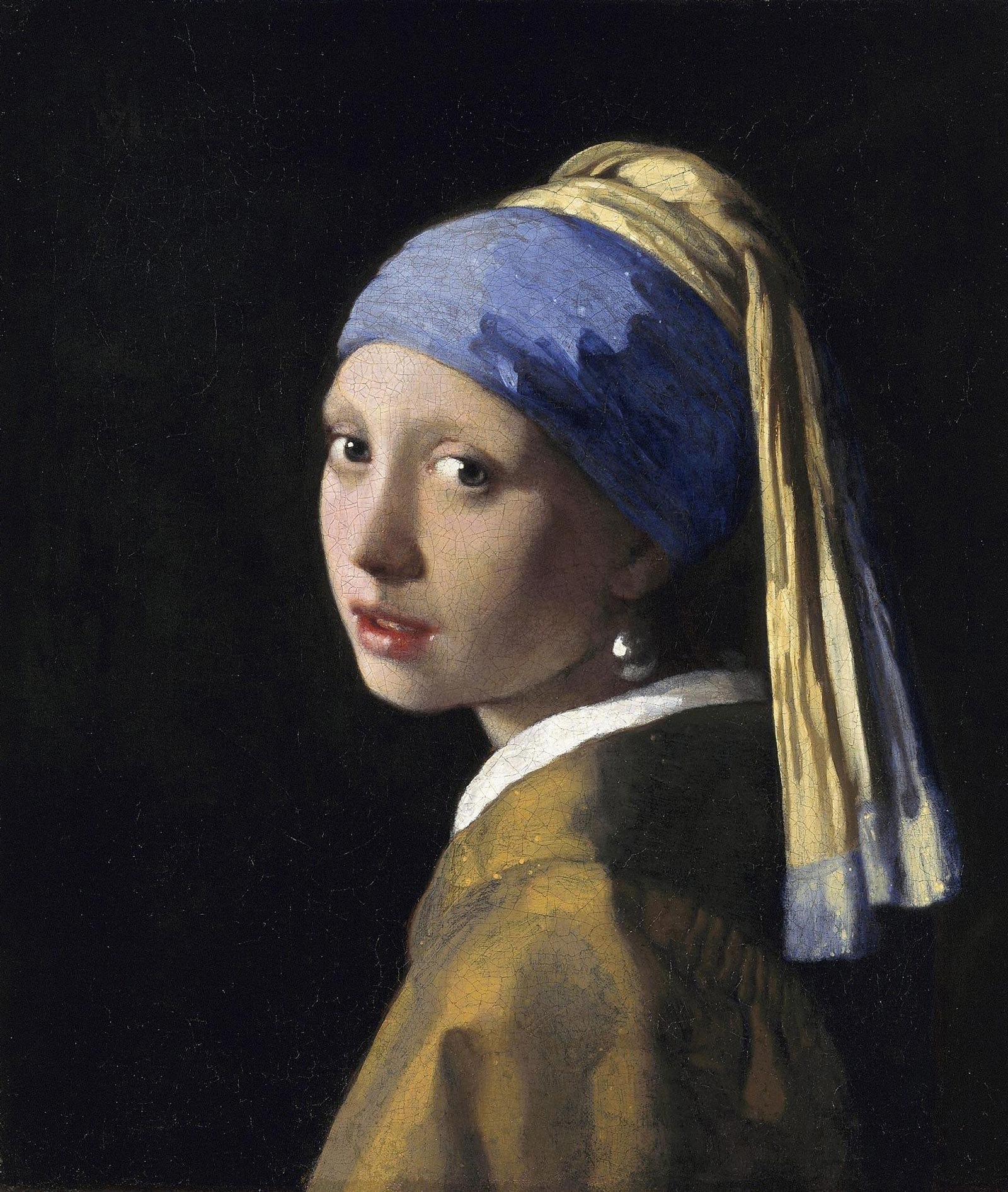This detailed painting, titled "Girl with a Pearl Earring" by Vermeer, depicts a young woman in a three-quarter profile against a dark background. She has brown eyes and light pink lips, with her head subtly turned towards the viewer. Her attire includes a bulky golden-colored top with a white collar and subtle dark brown shading. The lower part of the garment continues this intricate coloration. She sports a distinctive blue and yellow head wrap: the blue fabric surrounds her forehead like a thick headband, transitioning into a yellow knot that drapes down her back, resembling the form of a ponytail. A single, shimmering pearl earring dangles from her left ear, catching the light. This classical image, devoid of any text, other figures, animals, or buildings, emphasizes the subject's serene, contemplative expression.